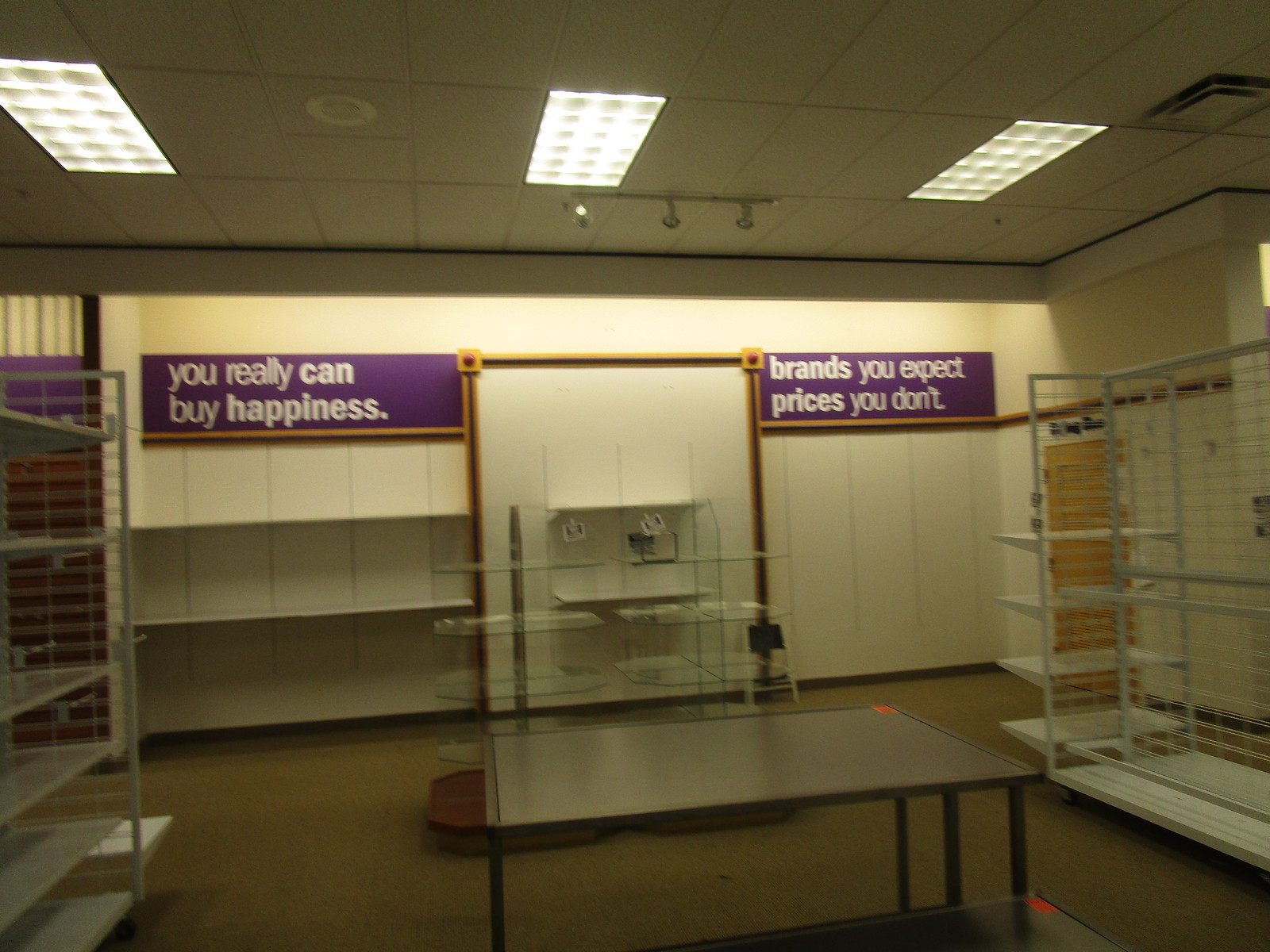The photograph depicts an empty storeroom with a few remaining pieces of furniture and fixtures. The room is dimly lit by three overhead fluorescent lights and three track lights mounted on a typical office drop ceiling with white, rectangular tiles. On the back wall, two purple signs with white lettering are prominently displayed. The sign on the left reads "you really can buy happiness" with the words "can" and "happiness" in bold, underlined by a gold bar. The sign on the right says "brands you expect, prices you don't," with "brands" and "prices" bolded, and is separated from the first sign by a yellow bar.

White shelving units are present along the left and right sides of the room, with additional glass shelves in the center. A dark brown coffee table with a hot pink tag sits in the foreground, alongside another dark table, also featuring a pink tag. The floor is tan in color. The architectural elements and decor of the room, such as the white or very light cream-colored walls, create a stark contrast to the empty space and give the storeroom an unfinished, transitional appearance.